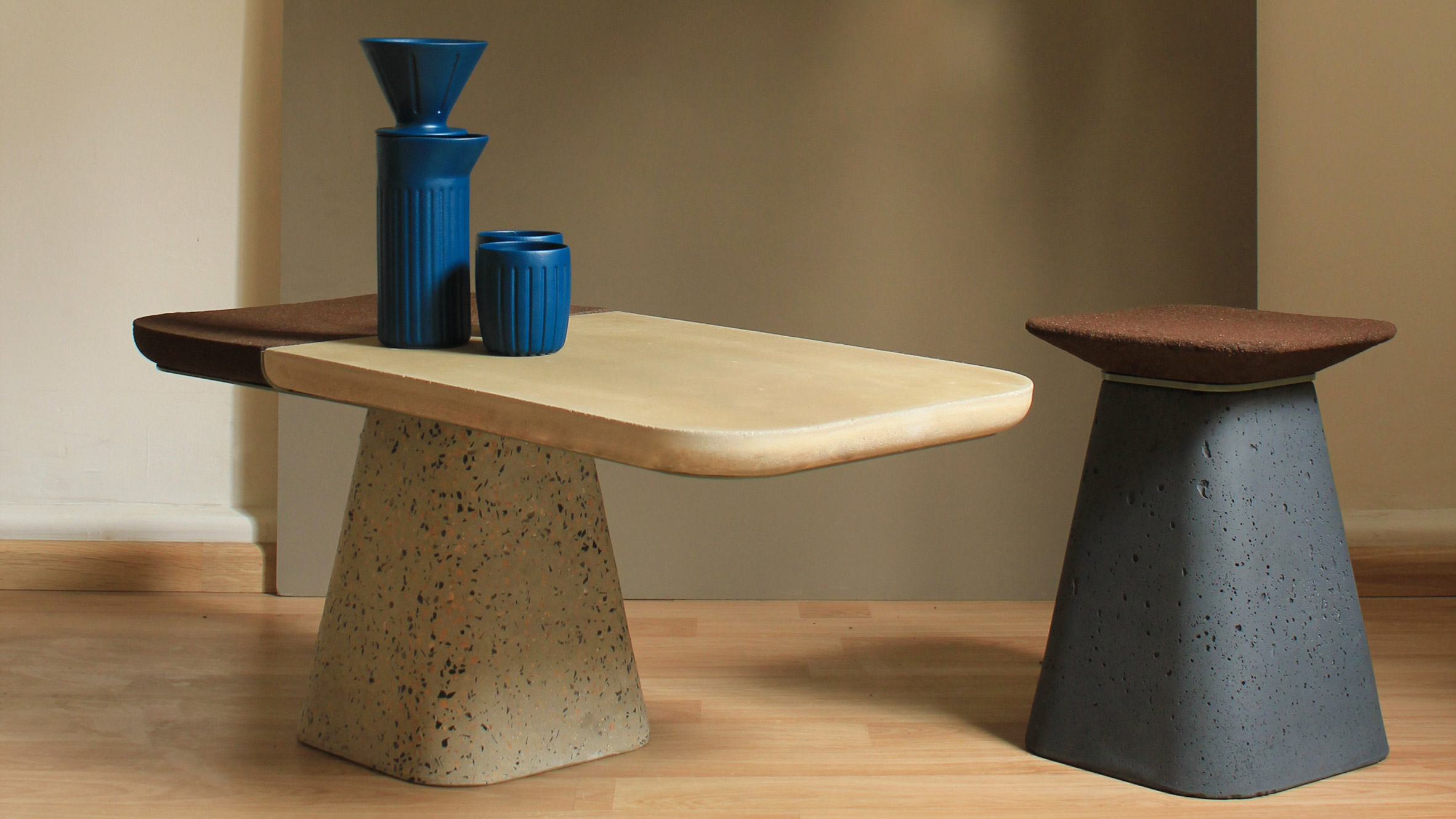In the image, two truncated pyramid-shaped stone objects are depicted, with the base wider than the top. The left stone is a light sandy color with dark speckles, possibly made from porous concrete. Atop this stone is a two-toned wooden cutting board—smoothly sanded, it features a light-colored front and a dark brown back. Above the board, two blue cups and a matching blue decanter are placed, possibly suggesting a tea or sake setting. Adjacent, to the right, is a gray stone object with a wide, flat, reddish-brown square surface on top, which might serve as a seat or a tabletop. The background showcases a metallic surface above a white wall, adorned with wooden trim at the bottom. The objects rest on a light hardwood laminate floor, creating a striking contrast with the stone materials.